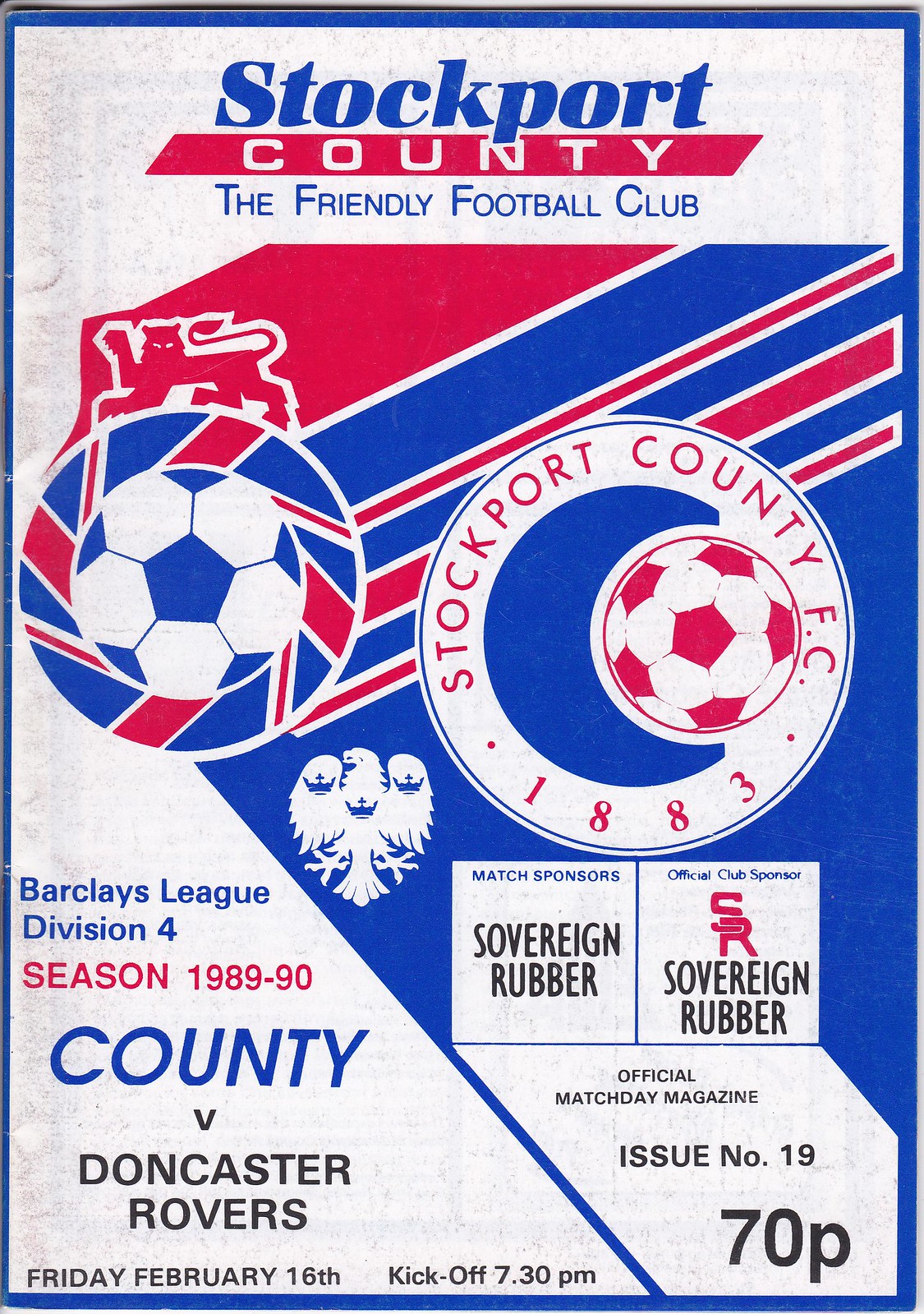The image depicts the cover of an official matchday magazine of Stockport County Football Club, also known as "the Friendly Football Club." The cover prominently features the club's logo: a blue circle with a soccer ball and the year 1883, surrounded by red text. The cover is mainly white with red and blue text and design elements. The magazine is issue number 19 and is priced at 70 pence. It includes details about a match in the Barclays League Division Four for the 1989-1990 season, specifically between Stockport County and Doncaster Rovers, scheduled for Friday, February 16th, with kickoff at 7:30 p.m. The match sponsor and the official club sponsor are both Sovereign Rubber. The cover also features the Stockport County emblem, which includes eagles and crowns.